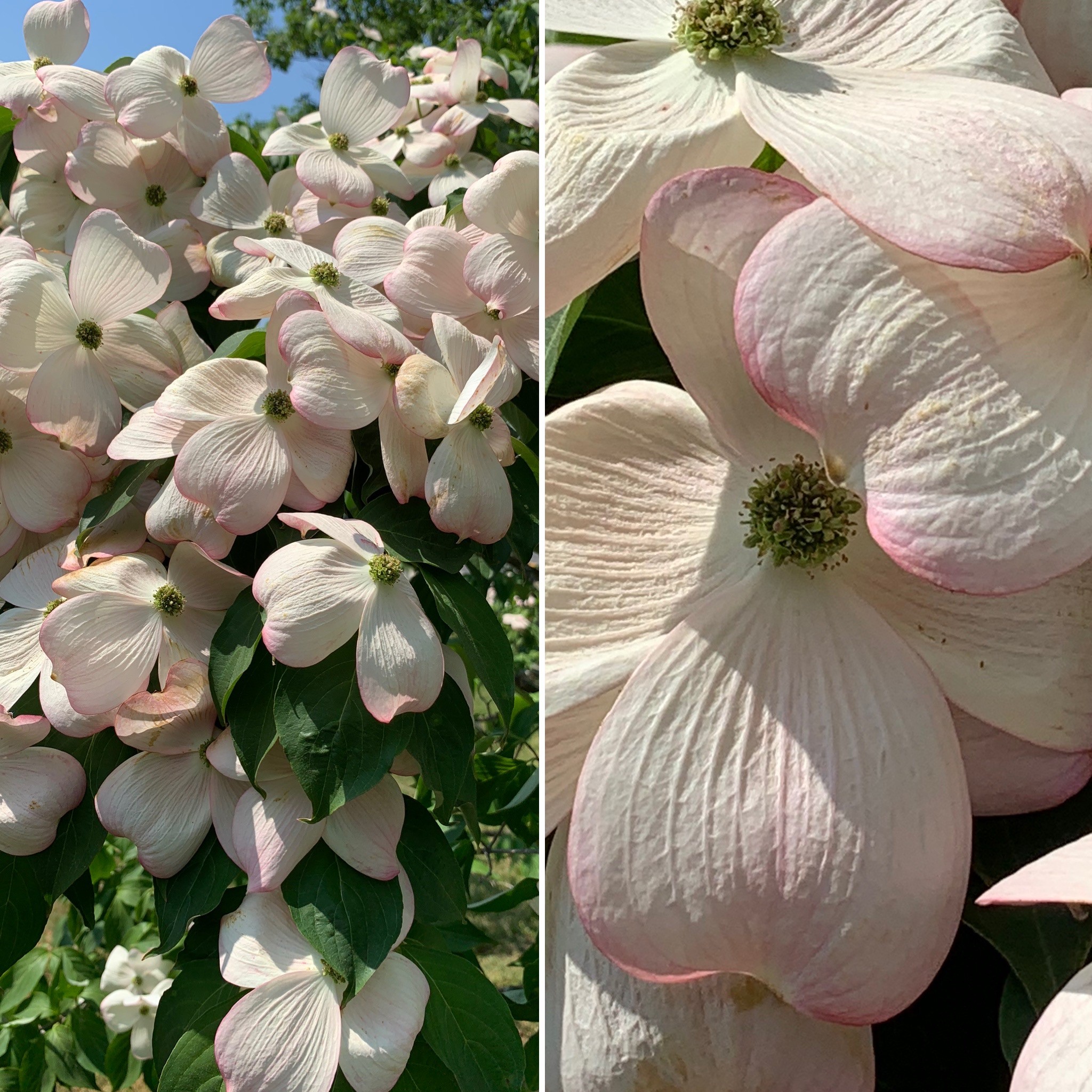The image consists of two side-by-side color photographs of densely packed flowers with white petals tinged with shades of pink. The first photograph on the left shows a cluster of these blossoms, likely magnolias or gardenias, layered densely with vibrant green leaves peeking through. In the background, a taller tree extends upwards with a sliver of light blue sky visible in the upper left corner. The sunlight catches on the petals, enhancing their delicate texture.

The second photograph on the right offers a close-up view, focusing on the intricate details of the petals and their pale pink to dark pink edges. The close-up reveals the green and yellow pollen in the center, with at least three or four blossoms overlapping each other, showcasing the same flowers as the wider shot. The detailed shot emphasizes the gentle, dainty quality and texture of the petals, highlighted by the subtle interplay of light.